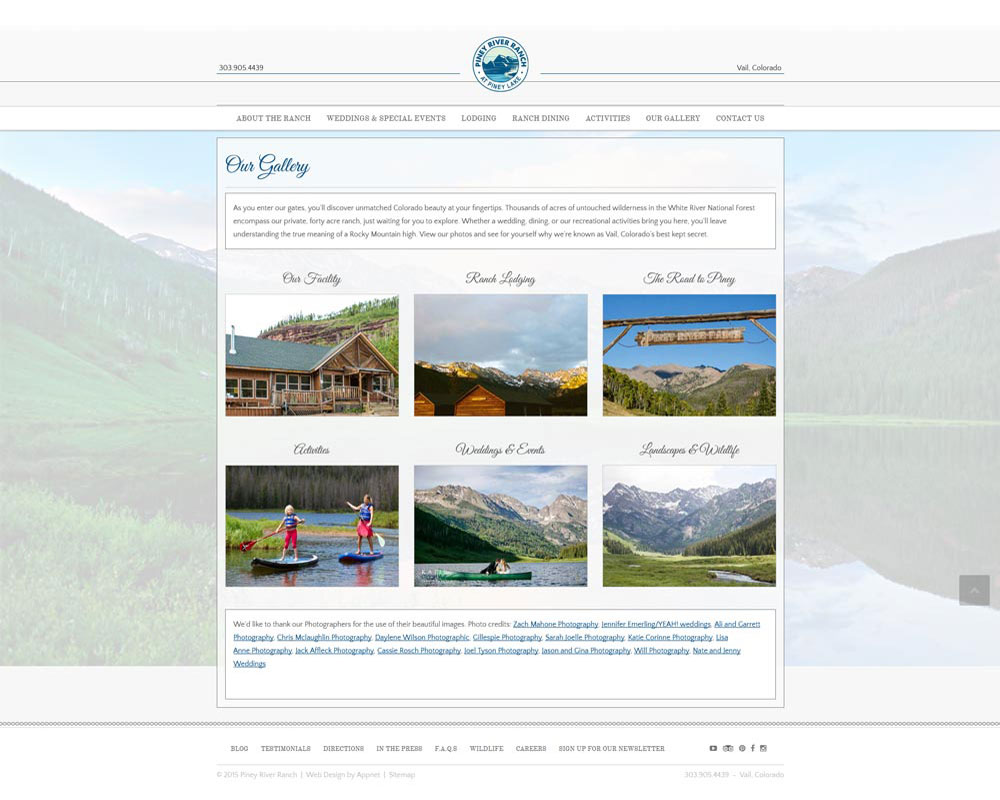**Screenshot of a Gallery Website**

The website appears to be a gallery showcasing various aspects of a facility. The gallery is organized into two rows, each containing three images with descriptive labels above them.

**Top Row:**
1. **Our Facility:** The first image on the top left features a sprawling log cabin-style building with a green roof. The structure is long and made entirely out of wood, giving it a rustic and inviting appearance.
2. **Ranch Lodging:** The middle image presents a picturesque, outdoorsy setting, indicative of a ranch. This likely showcases the accommodation options available at the facility.
3. **The Road to [Illegible]:** The third image features a sign marking the entrance to the facility. The exact wording on the sign is unclear, but it serves as a welcoming point for visitors.

**Bottom Row:**
1. **Aesthetics:** The first image on the bottom left highlights two people standing and rowing on kayaks, showcasing the recreational activities available and the natural beauty of the surroundings.
2. **Weddings and Events:** The middle image suggests that the facility is a venue for weddings and other significant events, indicating a picturesque and accommodating setting.
3. **Landscape and Wildlife:** The last image celebrates the natural beauty and wildlife that can be found at the facility, perhaps illustrating serene landscapes and native fauna.

Overall, the gallery effectively depicts the diverse features and attractions of the facility, ranging from accommodations and aesthetics to event hosting and natural landscapes.